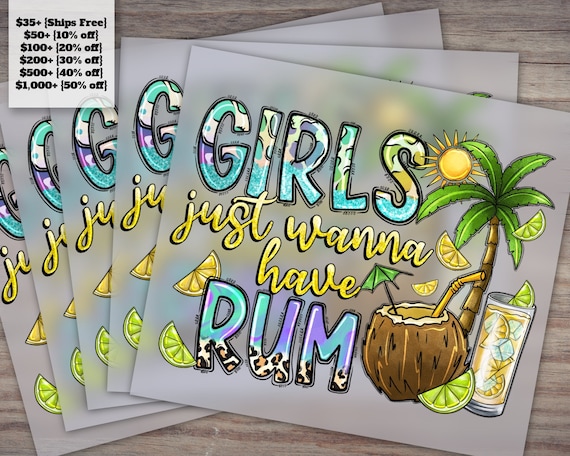This vibrant advertisement showcases a set of five party invitations stacked in a fan-like arrangement, each vividly designed with the phrase "Girls Just Wanna Have Rum." The words "girls" and "rum" are rendered in bold, block letters featuring a playful watercolor effect with hues of blue, green, and yellow, complemented by a stylish cheetah print at the bottom half of "rum." The phrase "just wanna have" is presented in a bright yellow font, adding to the tropical feel. Scattered across the vibrant backdrop are illustrations of lemons and limes, enhancing the festive summer theme. The right side of the image features detailed depictions of a sunny tropical scene, including a palm tree, a sun, a coconut with a straw and umbrella, and a tall glass filled with a drink, ice cubes, and citrus slices. These elements are set against a rustic grayish-brown wooden background, adding a natural touch. The upper left corner prominently displays pricing details, indicating free shipping for orders $35 and up, and escalating discounts up to 50% off for orders of $1,000 or more. This colorful and detailed layout combines text and tropical visuals to create a lively and inviting promotional piece.